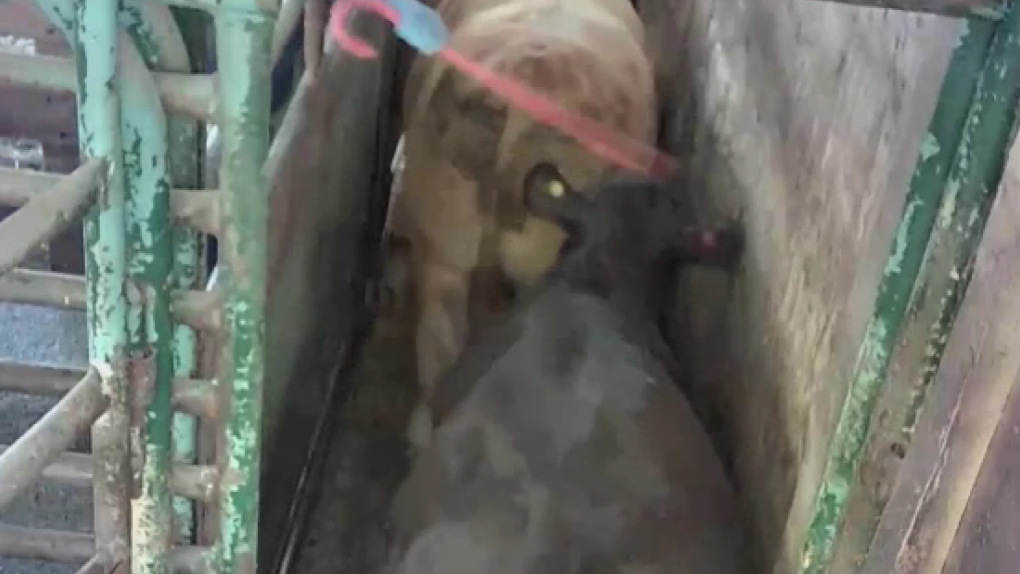The image is a close-up, blurry photograph capturing a scene with two cows inside a crate-like structure. The first cow, tan in color, is positioned in front, with only its backside visible. The second cow, which is darker brown, has its front and middle part visible. The crate has metal bars with vertical and horizontal crossbars on the left side, while the right side features a concrete wall with faded green vertical bars. A hand is seen maneuvering a red cane-like object, possibly a hook or a bar, towards the second cow, seemingly encouraging the cows to move forward in the tunnel-like space. The entire image has a sense of motion and indistinctness, particularly around the cane, indicating movement.